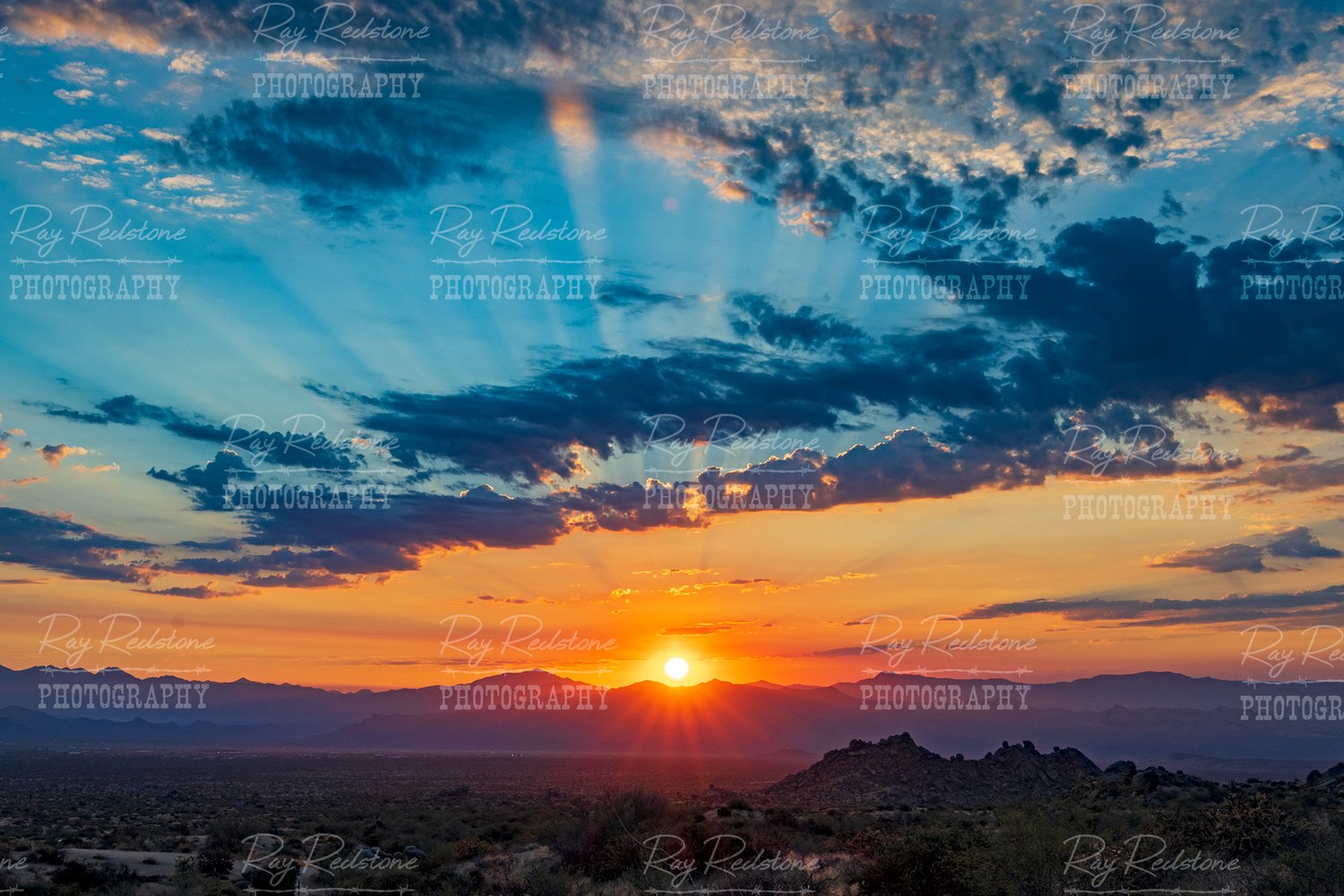The image captures a mesmerizing scene, likely showcasing either a sunrise or sunset. At the bottom, a brilliant white ball of the Sun dominates, surrounded by a plethora of radiant rays that streak across the sky. The background is painted in a gradient of warm hues, transitioning from deep oranges and reds near the horizon to a serene blue as the sky ascends. Scattered throughout are dark blue clouds, tinged with orange near their bases where they are kissed by the Sun's light.

Beneath this spectacular sky, a rugged landscape unfolds. A majestic, purple-hued mountain range lies directly below the Sun, contrasting sharply with the greenish mountains situated closer to the foreground. 

The entire image is overlaid with a semi-transparent watermark, repeating the text "Ray Real Stone Photography" in an elegant cursive script, ensuring credit is clearly given to the photographer.